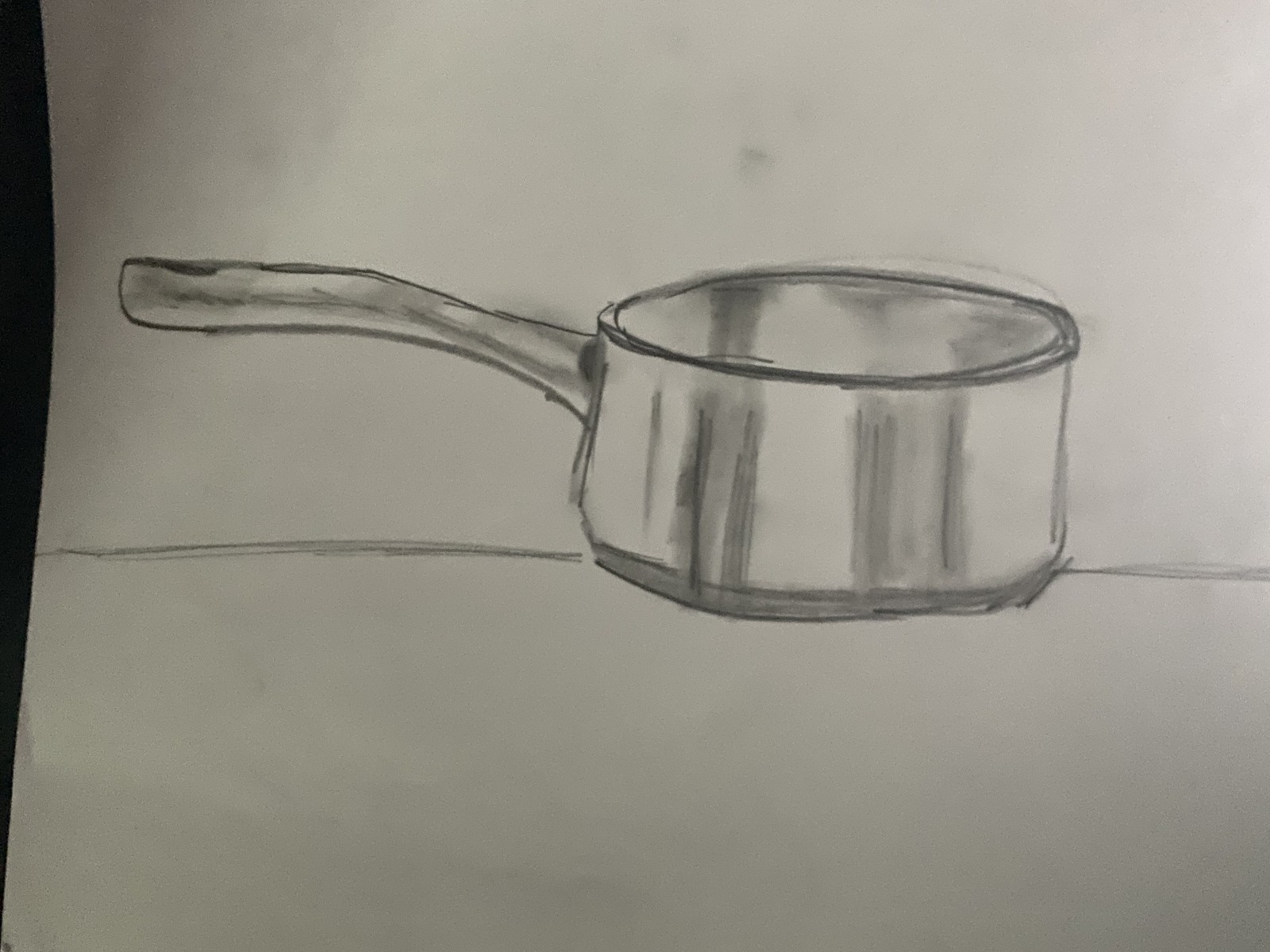This is a detailed hand-drawn image of a pot, created using a combination of crayons and colored pencils. The artist has employed shading techniques to give the drawing depth and dimension. The pot features a handle extending to the left from its base. It rests on a straight horizontal line, simulating the appearance of sitting on a table. The pot is rendered with a thicker outline for emphasis, and intricate shading is applied to the front, the handle, and the interior, enhancing the three-dimensional effect and giving it a realistic look.